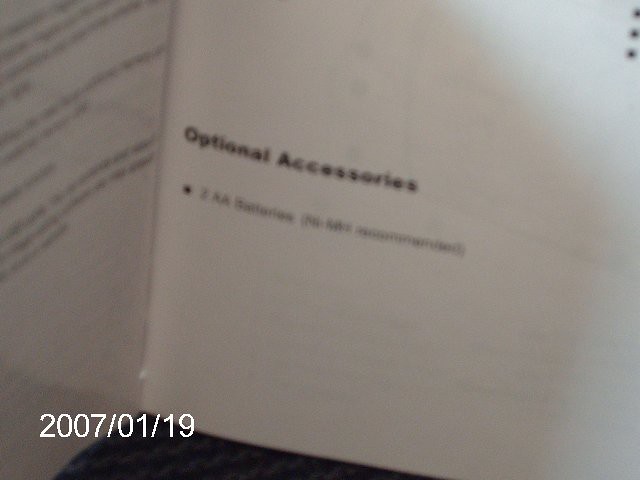This slightly horizontal image captures an open instruction manual of an unspecified device. The left-hand page, angled outward from the binding towards the lower left corner, features small black text on a white background. 

A date stamp in white reading "2007-01-19" appears prominently on this page. The right-hand page, visible from the middle downward, has a heading in bold black letters that states "Optional Accessories." Below this title, there is information pertaining to AA batteries.